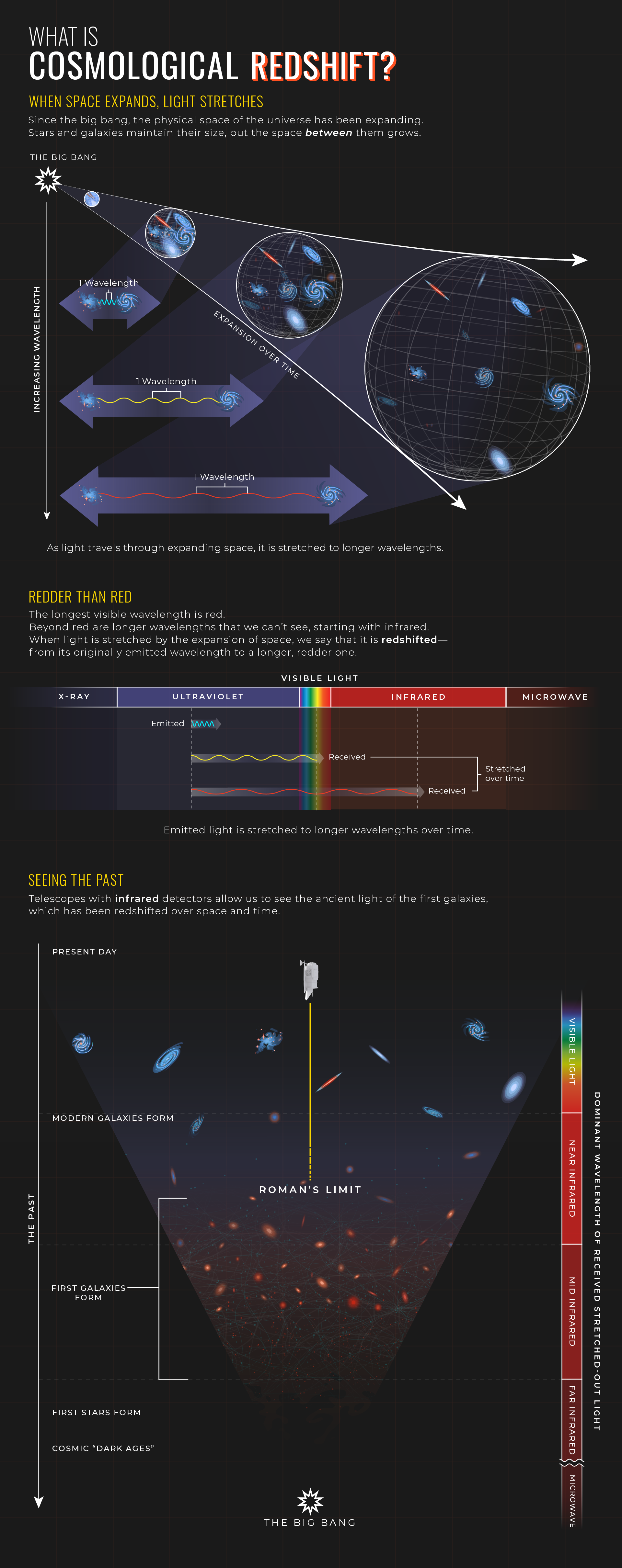The infographic, titled "What is Cosmological Redshift?", is presented on a solid black background. The primary focus is to explain the concept of redshift, where it states, "When space expands, light stretches." This idea is visually supported by a series of diagrams and images.

At the top left, a sequence from the Big Bang to the present day is illustrated through three expanding circular shapes that denote the universe's expansion. A line indicating "increasing wavelength" and another line labeled "expansion over time" show the stretching of light waves as space grows. One diagram explicitly addresses "redder than red," explaining that as light travels through expanding space, it stretches to longer wavelengths, transitioning from visible light into the infrared spectrum.

The infographic includes visible light as a rainbow, flanked by sections of electromagnetic spectrum: X-ray, ultraviolet on one side, and infrared, microwave on the other. A detailed visual comparison shows light received today against the same light stretched over time into the red and infrared wavelengths.

The timeline diagram below traces the history of the universe from the Big Bang at the bottom to present-day modern galaxies at the top. Key points such as the formation of the first stars, the cosmic dark ages, and the emergence of the first galaxies are marked. The conical shape visualizes this progression, with the present-day visible light shown near the top, and the increasingly redshifted ancient light towards the bottom.

Additionally, a visual representation of redshift shows three circles (small, medium, larger) depicting expanding space with arrows pointing outward. Another diagram, resembling a V-shape with red and blue dots, likely represents the shift in spectral lines due to redshift.

Overall, the poster functions as an educational tool, likely intended for school use, to graphically illustrate how the universe's expansion affects light over time, making distant galaxies observable in the infrared spectrum with telescopes. The blend of clear visuals and annotated diagrams effectively conveys the essence of cosmological redshift to viewers.